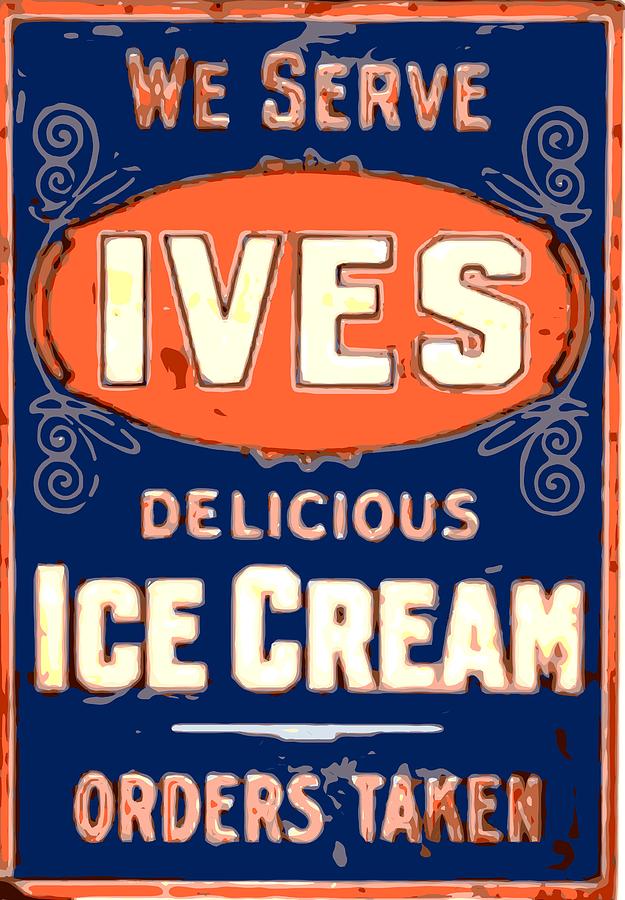The image depicts an old metal sign with a dark blue background and an orange border adorned with red dots. At the top of the sign, in all capital letters, it reads "WE SERVE" in slightly distorted orange text. Beneath this, there is a large, circular, egg-shaped orange section that contains the word "IVES" in white block letters, though the letters appear slightly stained yellow. Flanking the circular section are intricate flowery, curly designs. Below "IVES," the word "DELICIOUS" is written in all caps with slightly distorted pale orange letters, followed by "ICE CREAM" in stained white block letters with hints of light orange. At the bottom of the sign, it states, "ORDERS TAKEN" in the same pale orange text as the previous lines. The sign is designed vertically and is brightly lit, showcasing its nostalgic charm.